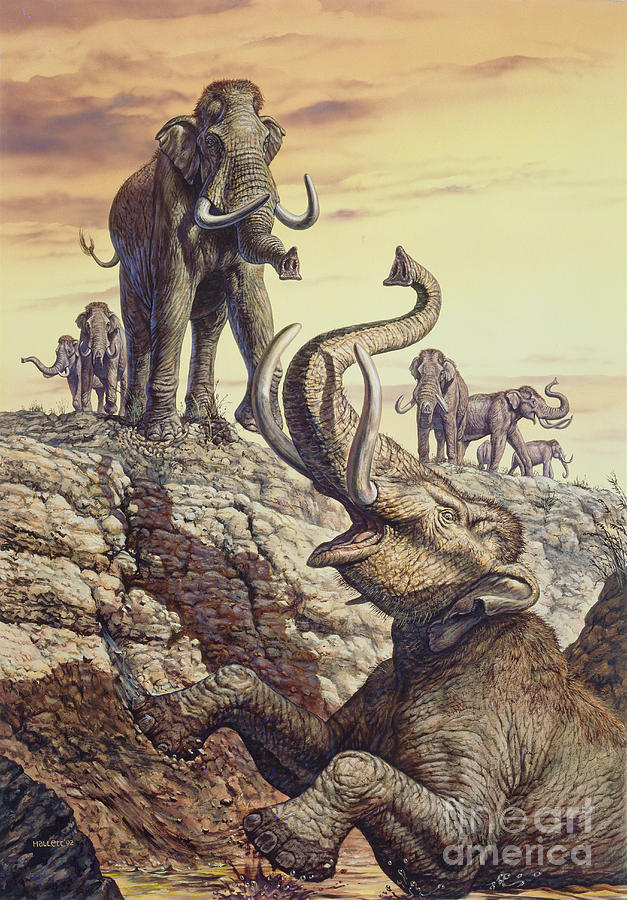The image showcases a stunningly realistic and detailed illustration with a watermark that reads "Heart America." Dominating the foreground is a large elephant standing on its hind legs in a water hole, its front legs lifted, trunk curved upward in an S-shape as it trumpets with its head raised and mouth open, revealing its two ivory tusks. Surrounding this water hole is a cliff composed of brown, gray, and tan colored rock. Atop this cliff is a second elephant, facing the trumpeting one directly, standing on all fours with its tusks clearly visible. In the background, a group of six elephants, of varying sizes, can be seen amidst the rocky landscape. Some have their tusks raised while others have them relaxed, seemingly foraging. The entire scene is bathed in the warm hues of a watercolored sunset that transitions from yellow and orange to reddish and purplish tones, adding to the prehistoric feel of the illustration.